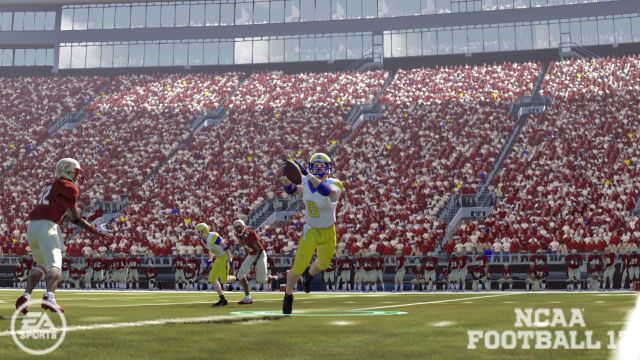In this screenshot from an EA Sports NCAA Football game, the central action features a thrilling moment as a player in a white jersey with a yellow number 8 and matching yellow pants catches the football mid-field. Surrounding him are players from both teams, with notable interactions including a teammate and an opponent—dressed in red jerseys with white pants—engaged in a dynamic contest. One red team player, specifically wearing number 42, stands slightly to the left, monitoring the play. 

This virtual stadium, depicted in the upper section of the image, reveals box seats adorned with silver trim along the bottom barriers. The windows of these seats reflect the light, obscuring any view inside. Beneath these seats, the crowd's energy is palpable, a sea of red and white jerseys representing the home and visiting teams. On the sideline, the red team is lined up, emphasizing their presence just below the enthusiastic audience. The detailed environmental and character designs enhance the immersive experience of this electronically simulated football game.